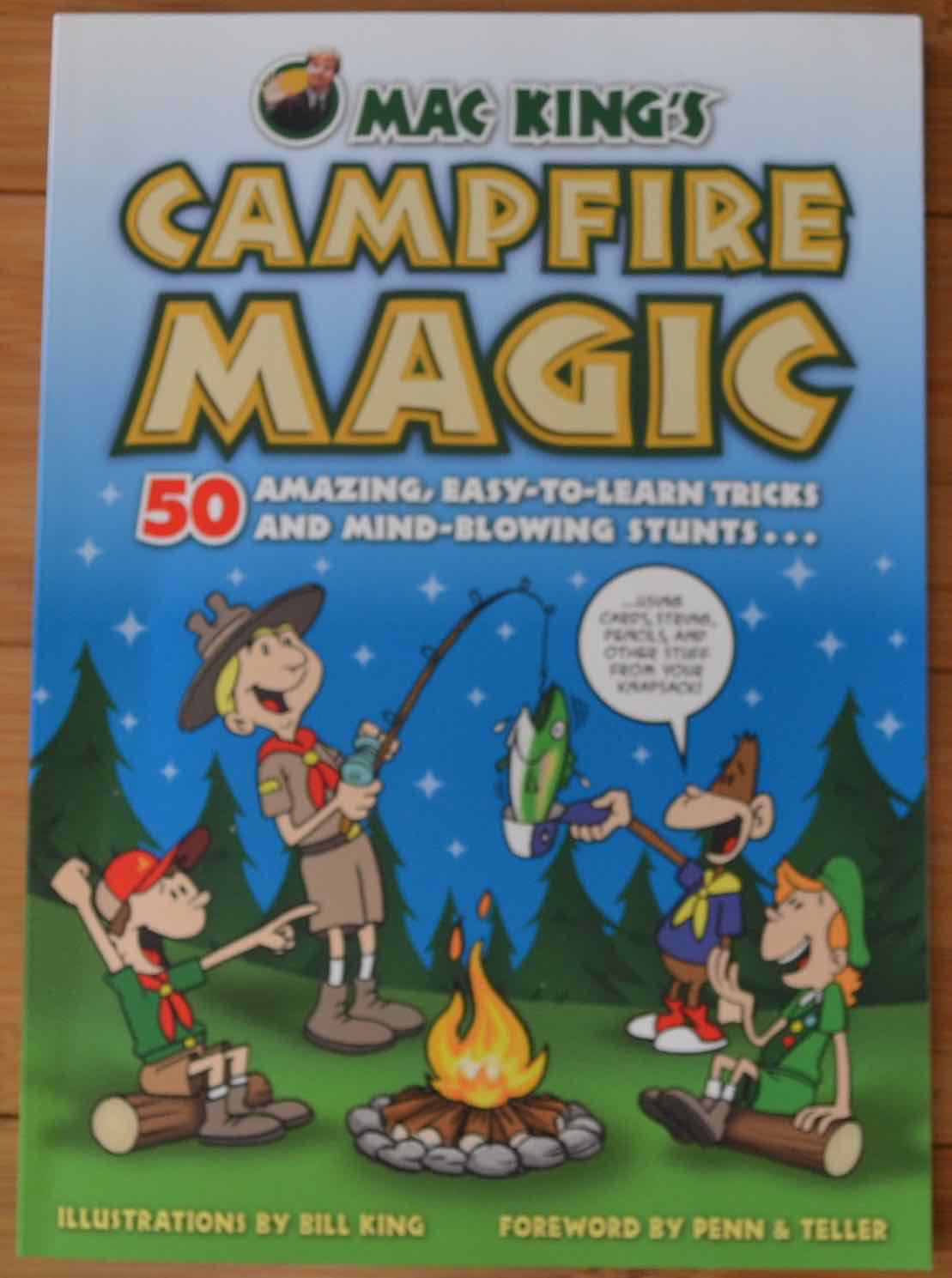The cover of the children's book "Mack King's Campfire Magic" is prominently displayed against a wooden surface. The background of the cover transitions from light blue to dark, providing a captivating backdrop. "Mack King’s" appears in a green font, accompanied by a circle on the left showcasing Mack King's face. Just below, "Campfire Magic" is written in yellowish lettering bordered by green. The tagline underneath reads, "50 Amazing Easy-to-Learn Tricks and Mind-Blowing Stunts." Illustrated by Bill King with a foreword by the famous magicians Penn & Teller, the scene on the cover features several characters around a campfire: Mack King, wearing a Boy Scout-like uniform, two Boy Scouts, one Girl Scout, and a playful monkey sporting a yellow neckerchief. The monkey holds a cap with a fish, while a Boy Scout uses a hook to fish over the campfire. The vibrant colors range from brown, white, black, yellow, green, orange, and purple, enhancing the lively atmosphere. The characters are centrally positioned, with text bubbles unreadable but contributing to the animated scene where they all sit on logs around the fire, laughing and engaging in campfire magic.